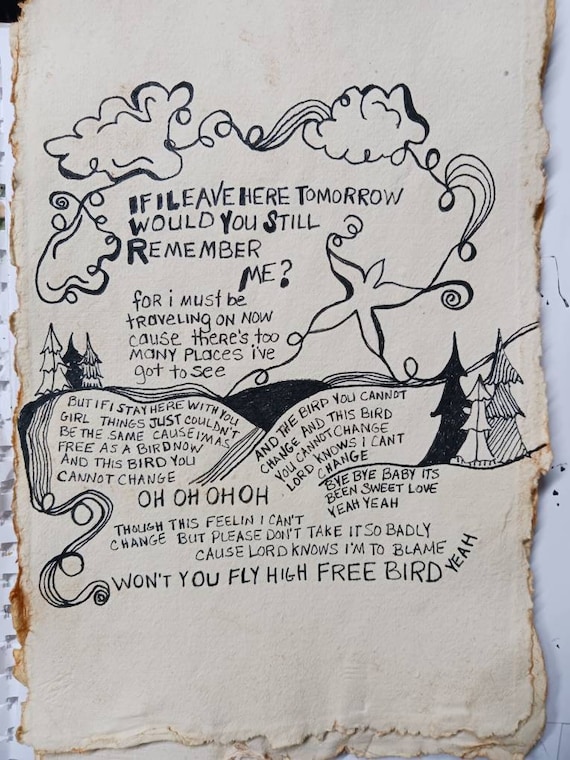The image is a color photograph of aged, tattered pages that appear to have been ripped from a journal. These off-white, worn pages are placed on top of a notepad. The edges are torn and frayed, adding to the old appearance of the paper. On these pages, there is a handwritten transcription of song lyrics, prominently starting with "If I leave here tomorrow, would you still remember me?" The text continues with lines like "For I must be traveling on now, because there are too many places I've got to see," and "But if I stay here with you, girl, things just couldn't be the same, because I'm as free as a bird now, and this bird you cannot change." The lyrics include repetitions such as "change, and this bird you cannot change" and additional phrases like "Lord knows I can't change, bye bye bye baby," "It's been sweet love, yeah I bet," and "won't you fly high, free bird, yeah."

The pages also feature several sketches, including wispy clouds, trees resembling Christmas trees, a leaf falling to the ground, and a star pattern forming an infinity loop. Additionally, there's a doodle of a mountain. All these illustrations are set against the textured backdrop of the journal pages, merging lyrics and art into a single evocative piece.